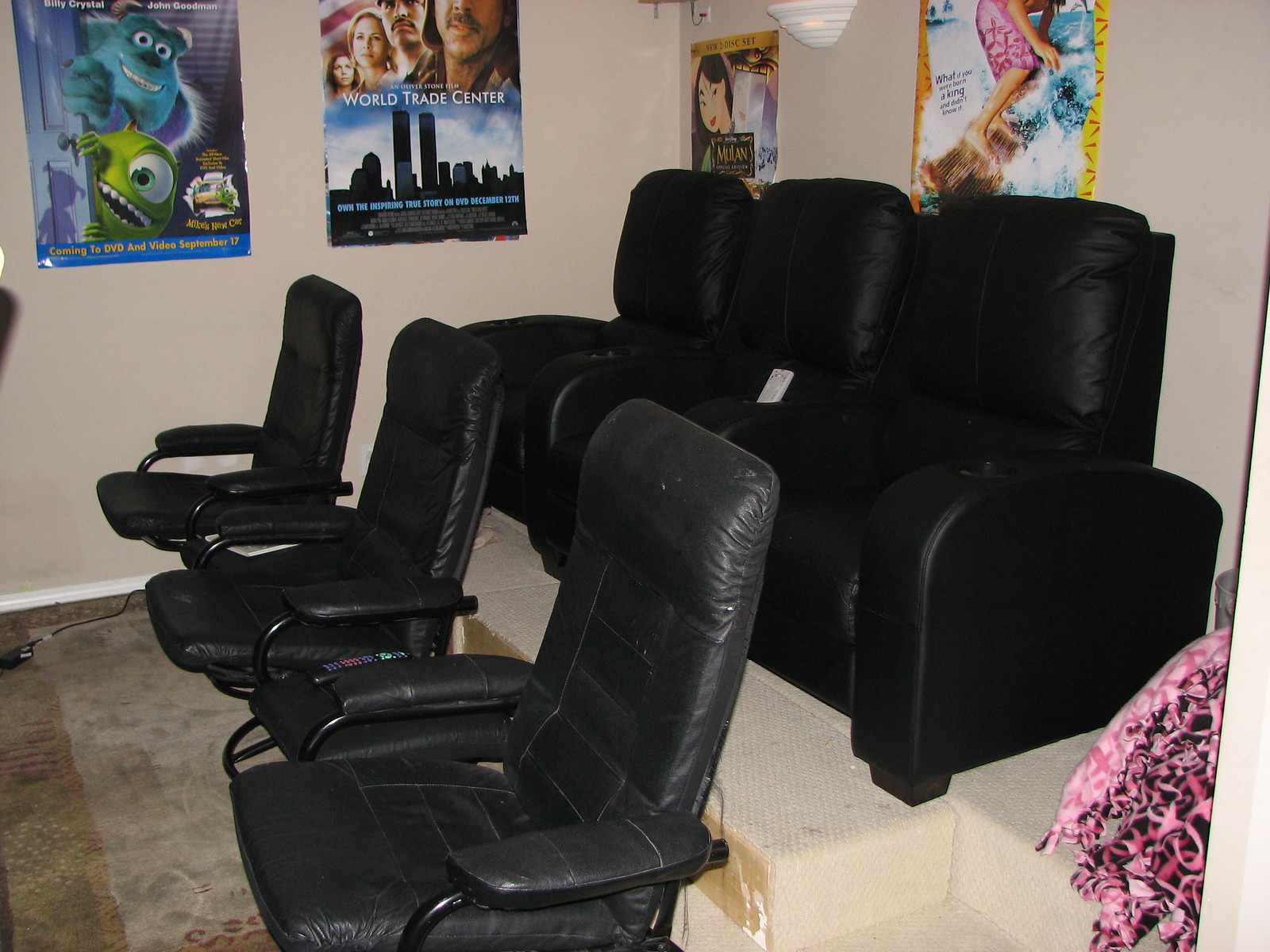The image features a cozy, small movie room with tan walls adorned with various movie posters, including ones for Mulan, Monsters, Inc., World Trade Center, and possibly Moana, with another poster depicting someone surfing. The room's seating consists of three large, black vinyl recliner chairs arranged on a raised platform, allowing for an elevated viewing experience. In front of these recliners, there are three black vinyl glider rockers positioned on a brown, intricately designed rug. A remote control rests against the back of the middle recliner, while another remote is on a table situated between the front two rockers. Additionally, a glimpse of something pink can be seen in the right corner of the room.